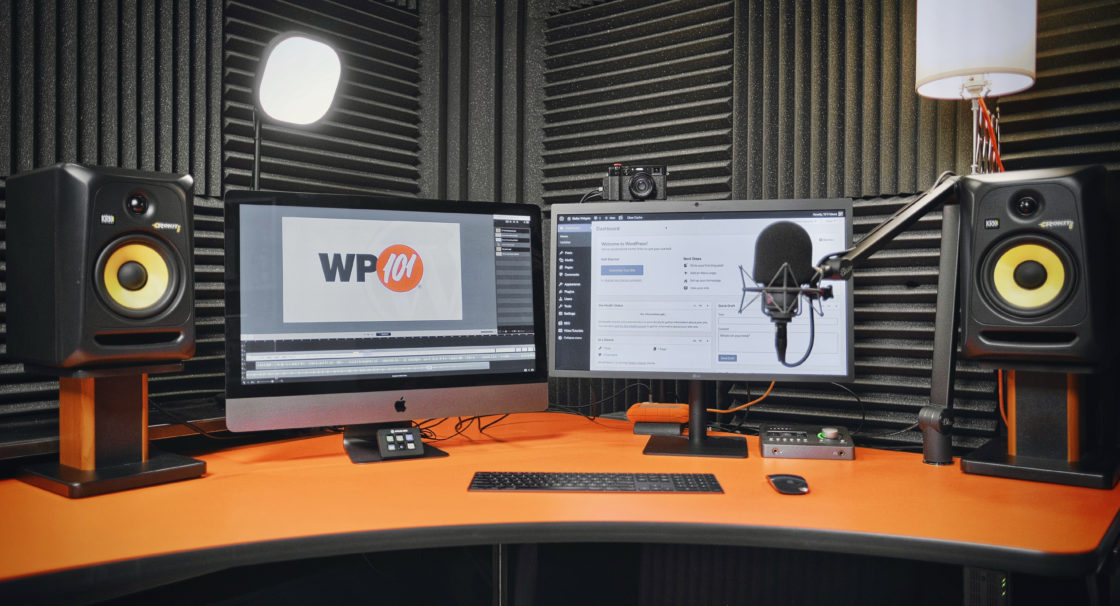The interior of a recording studio is showcased in this image, dominated by a large, orange corner desk at its center. The walls are lined with dark gray soundproofing panels, arranged in alternating vertical and horizontal patterns to optimize sound absorption. Both the desk and the equipment exhibit a professional setup, featuring two computer monitors flanked by raised speakers on either side. The left monitor displays the text "WP-101", likely the name of the station or studio. On the right, a white screen is visible. Suspended near the right speaker is an articulated arm holding a professional-grade microphone. A very flat keyboard and a wireless mouse rest on the desk, and a camera is perched atop one of the monitors. Illuminating the workspace, a light shines from the top of the left monitor, while another light is positioned near the right speaker. Various pads with buttons are scattered across the desk, though their functions are unclear from this vantage point.